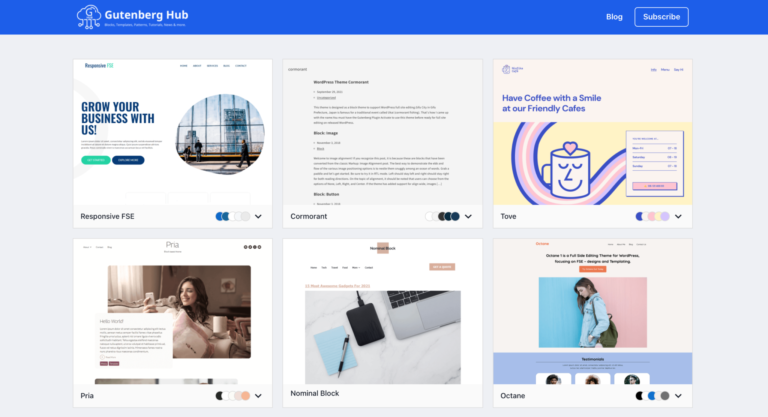A screenshot of the Gutenberg Hub interface is displayed. At the top, there is a blue bar with white text; on the right side of this bar, a blog link is visible alongside a subscription button. Below, six selectable boxes are arranged in a grid. The first box on the left, a white panel titled "Grow Your Business with Us" in blue text, features an asymmetrical circle with an image inside. This image shows a man walking down the street in front of a building, with two other people visible in the distance. The text "Responsive FSE" is positioned at the bottom of this box. Another box, on the far right, is labeled "Have Coffee with a Smile at Our Friendly Cafes." It includes a cartoonish illustration of a smiling coffee cup, complete with a heart above its head.